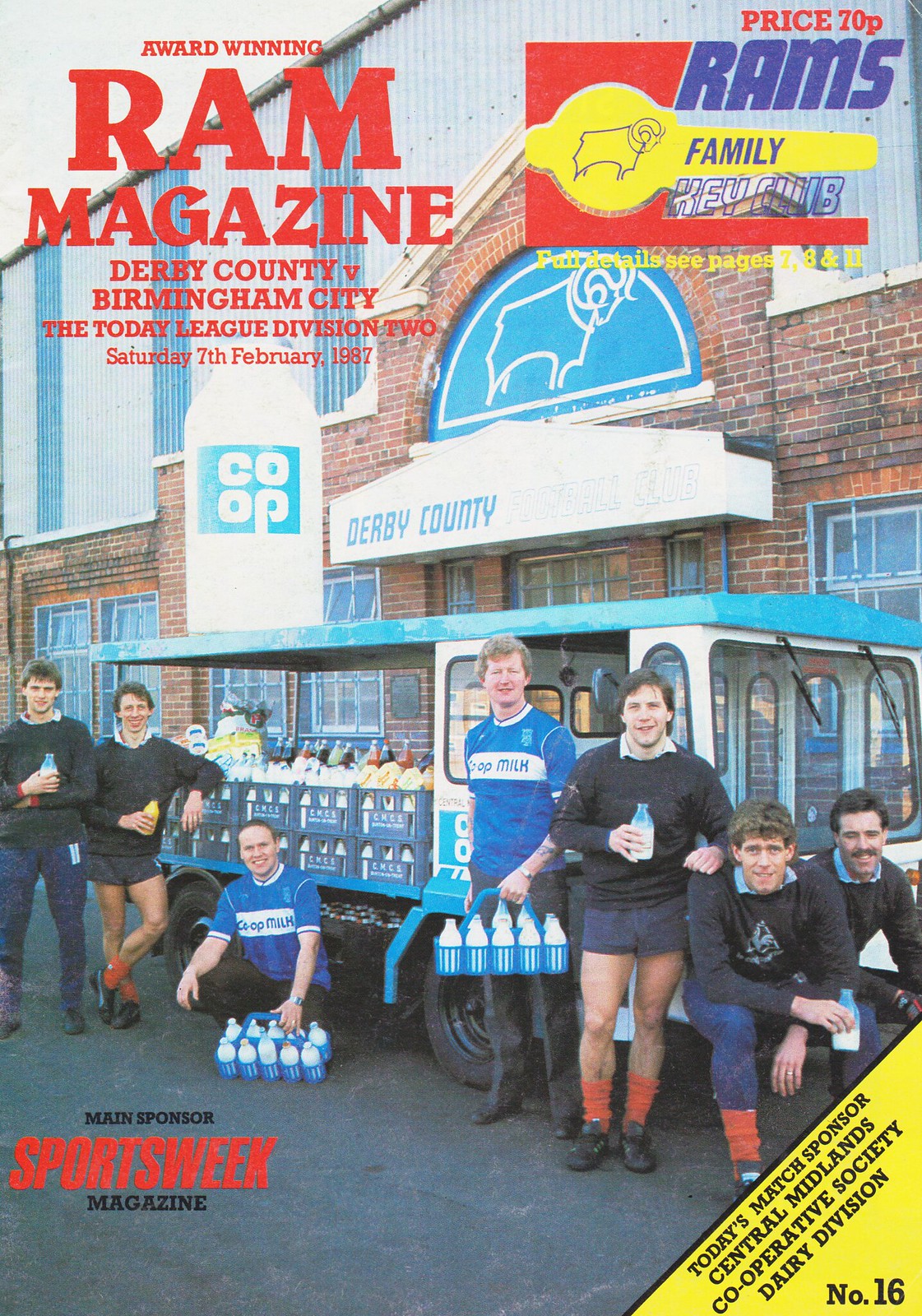The cover of the Award-Winning Ram Magazine features a vibrant scene set against the backdrop of a large stone building, adorned with a ram figure above the door and the name "Derby County Co-op." The focus is on seven young men, likely in their early 20s, posing in front of a vintage flatbed milk truck. The men, who appear to be athletes, are engaging with various milk beverages; some are sitting on the truck's bumper while others stand, holding either glass jars of milk or blue plastic milk holders, each containing ten milk jugs. One man leans on the truck with a bottle containing a yellow drink. The magazine highlights the Derby County versus Birmingham City match in the Today League Division II, which took place on Saturday, 7th February 1987. In the top right corner, it notes a price of 70P and mentions the Rams Family Key Club. At the bottom, the main sponsor is listed as Sports Week Magazine, and today's match sponsor is the Central Midlands Cooperative Society, Dairy Division, number 16.